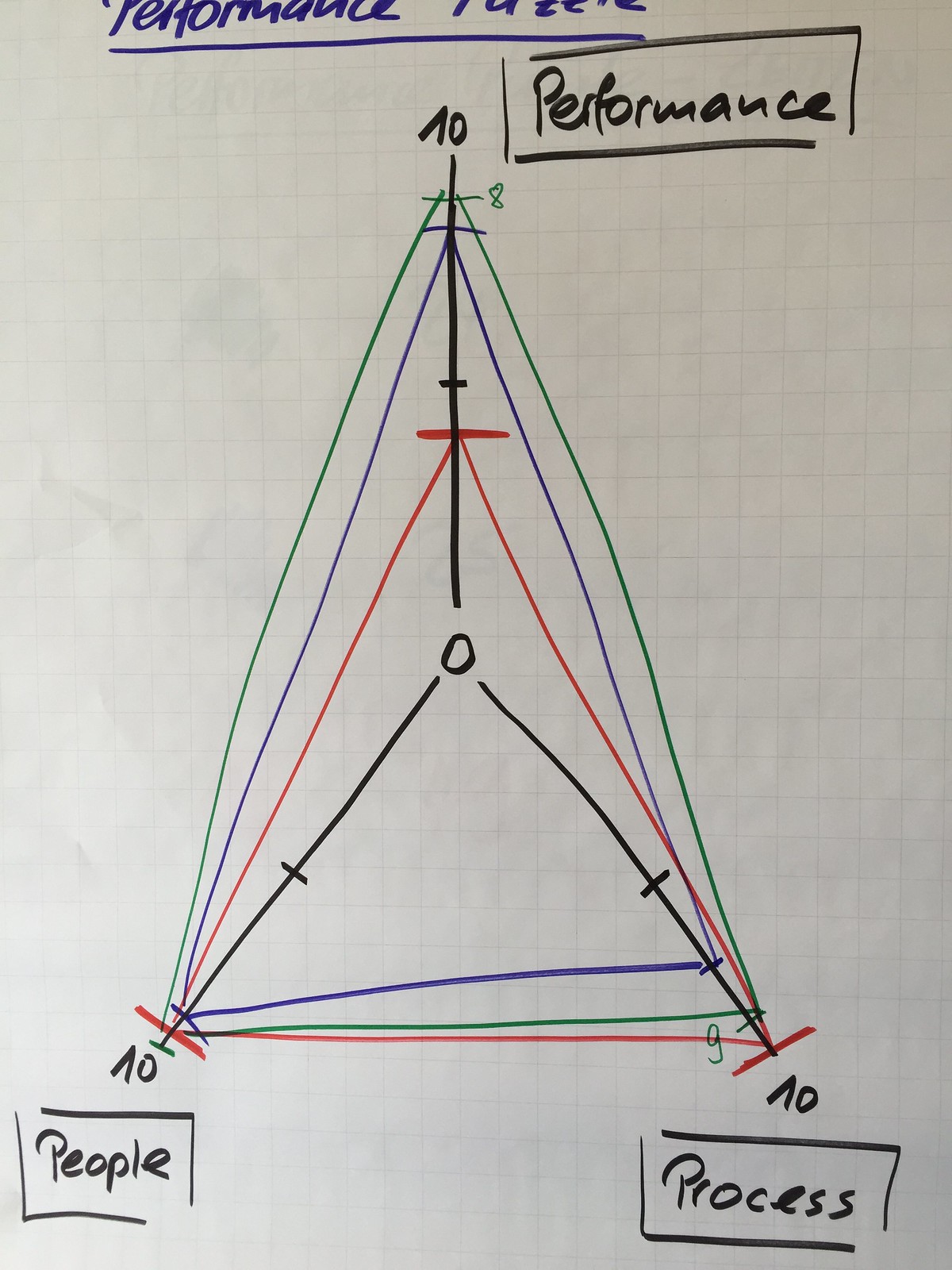The image features a graph arranged in a triangular layout. Three black lines converge at the center, each radiating outwards towards distinct labels in rectangular black borders. The top line points to the label "Performance," the bottom right line points to "Process," and the bottom left line points to "People." Interspersed along these lines are three differently-shaped and colored triangles, each representing various data points.

- The red triangle extends fully to the bottom but reaches only halfway up the central axis.
- The green triangle also reaches the bottom edges on both sides but extends predominantly towards the top.
- The blue triangle reaches fully to the bottom left, almost touches the top, and extends about two-thirds of the way along the bottom right.

Each triangle delineates varying extents to which performance, process, and people factors intersect, effectively visualizing the relationships and balance among these three critical elements.